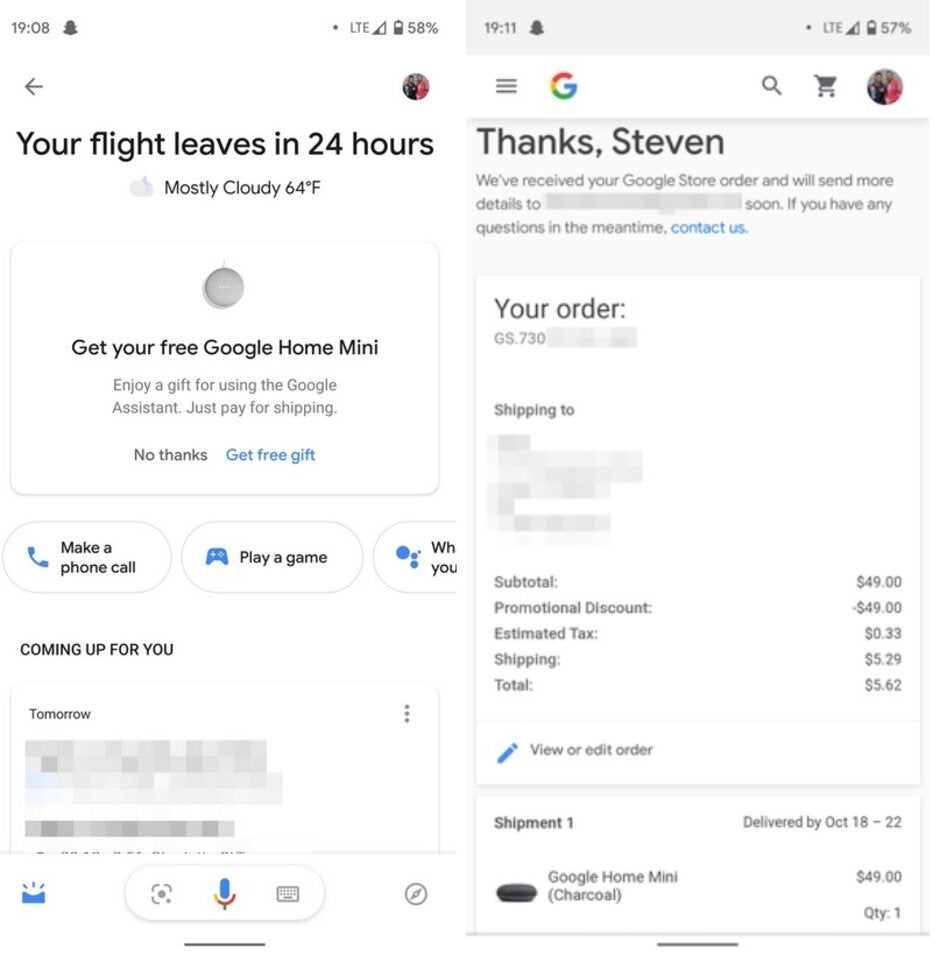The image comprises two vertically-aligned, side-by-side screenshots from a phone, which are vertical rectangles in shape. The upper portion of both screenshots features the standard phone menu.

The left screenshot contains a notification and is predominantly about an upcoming flight. An arrow pointing to the left accompanies the text, "Your flight leaves in 24 hours." Below this, a message reads, "Get your free Google Home Mini," followed by "Enjoy your gift," and "Coming up for you tomorrow." Additionally, there are links that prompt the user to play a game or make a phone call. The phone's voice command menu is visible on this side.

The right screenshot is a partially blurred email confirmation from the Google Store. This email starts with "Thanks, Steven," and continues, "We received your Google Store order and will send more details." The destination for the order is blurred out, but it states, "If you have any questions in the meantime, contact us." Details of the order include a subtotal of $49, a promotional discount of $49, a tax of $0.33, shipping cost of $5.29, and a total of $5.62, indicating the order of a free Google Home Mini. The order summary shows one charcoal-colored Google Home Mini, indicating a quantity of one, with expected delivery dates between October 18th and 22nd. The layout of the email is symmetrical and user-friendly.